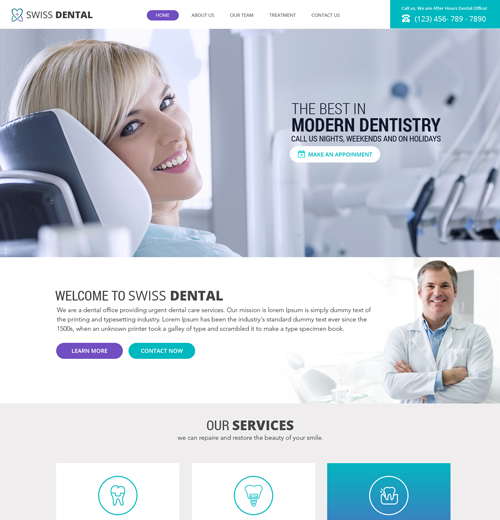This is a screenshot of the homepage of the Swiss Dental website. At the top, the header features the name "Swiss Dental" adorned with decorative hearts. Below this, a navigation menu with purple highlighting includes options for "Home," "About Us," "Our Team," "Treatments," and "Contact Us." 

In the top-right corner, there's a teal-colored box labeled "Call Us," although the text is blurry and unreadable. Next to it, a phone icon appears with the number "123-456-7890."

Central to the screenshot is an image of a woman sitting in a white and gray dentist chair, smiling. Adjacent to her image, text reads: "The Best in Modern Dentistry. Call us nights, weekends, and on holidays." A clearly visible button below this text says "Make an Appointment." To the right, dental equipment is noticeable in the background. The woman in the chair wears a blue shirt.

Below this section, there's a welcome message reading "Welcome to Swiss Dental," accompanied by information about the office. Two buttons beneath this message are in purple and green, labeled "Learn More" and "Contact Now," respectively.

To the left of this message is a photo of a smiling man with crossed arms, dressed in a white coat and blue shirt, evidently portraying the dentist.

Further down, a light gray rectangular box outlines their services and states, "Our Services: We can repair and restore the beauty of your smile." Under this box, three teal-colored icons are displayed: one of a plain tooth, one of a tooth with an unspecified object inside, and another of a tooth with a rectangular outline around it, which is highlighted in blue.